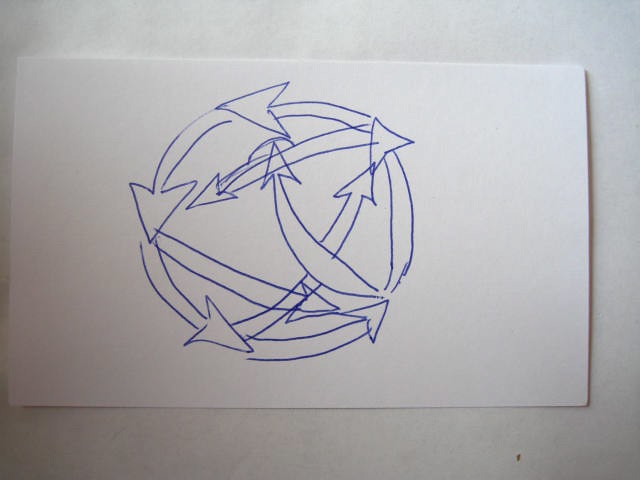A minimalist scene featuring a white background that could be either a tabletop or a wall, showcases a sturdy piece of cardstock at the center, distinguished from typical printer paper by its heavier weight and firm texture. The cardstock is adorned with a network of arrows, drawn in a bold, bubble-like style using a blue Sharpie. At the core, four arrows create a prominent circular formation. Among the surrounding arrows, one extends from the top left of the circle to the middle left, while another branches from the bottom right and moves straight upward. There’s a unique, dual-headed arrow crossing diagonally from the top right to the bottom left, and a nearly concealed arrow tracing a line from the top left to the bottom right, close to the circle’s border. Collectively, the disarray of arrows forms a chaotic yet intriguing pattern, suggesting a complex and perhaps nonsensical diagram.